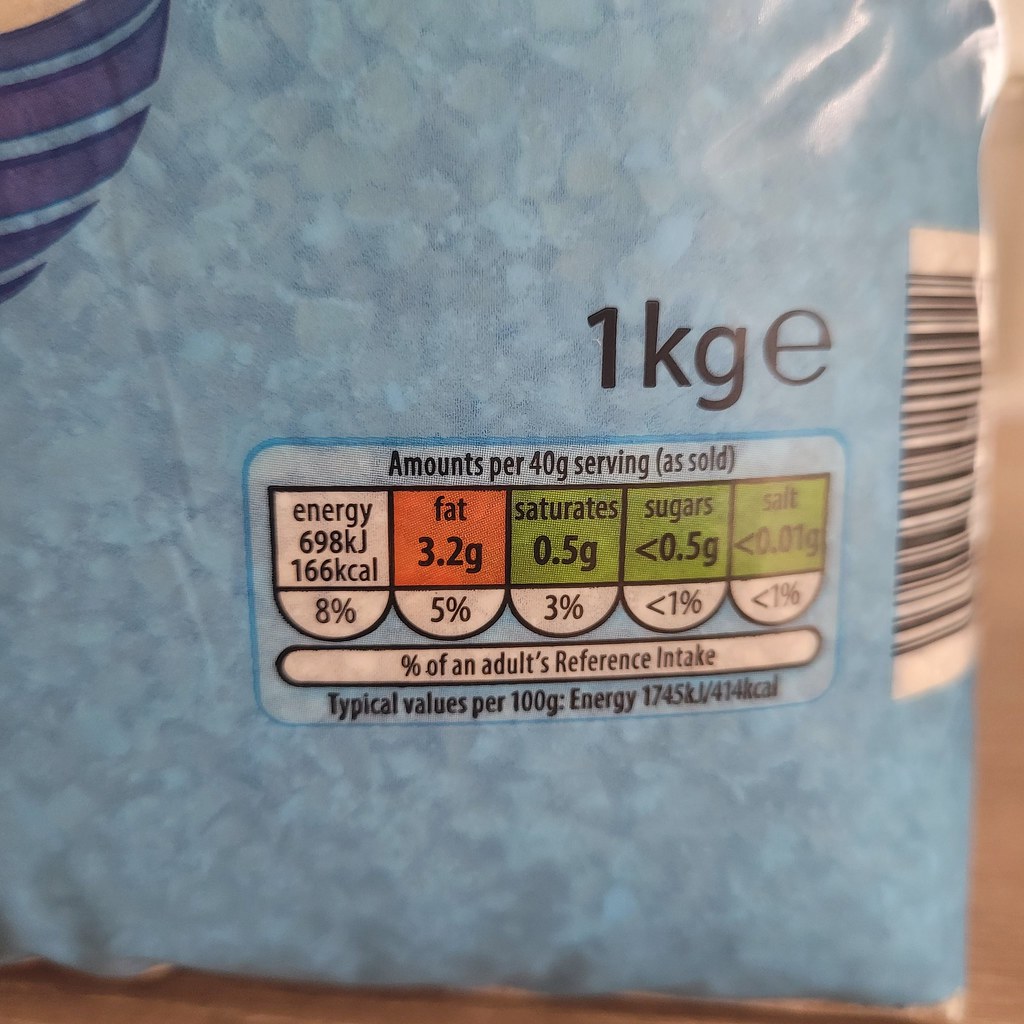This image shows a close-up of a plastic bag containing a clear, whitish crystal material, which appears bluish due to the shading of the bag. The bag is laying on a brown flat surface. In the upper left corner of the bag, there is a partially visible blue-lined globe icon. Prominently displayed on the packaging is the text "1 KGE" in large black font, positioned above a table that details nutritional information per 40 grams serving size. Blocks of color—white, orange, and three shades of green—highlight values for "Energy, Fat, Saturates, Sugars, and Salt" along with their corresponding amounts and percentages of an adult's reference intake. Specifically, the energy content is 698 kJ or 166 kcal (8%), fat is 3.2 grams (5%), saturates are 0.5 grams (3%), sugars are less than 0.5 grams (<1%), and salt is less than 0.01 grams (<1%). Further below, it states the typical values per 100 grams. A barcode is visible on the right side of the bag.